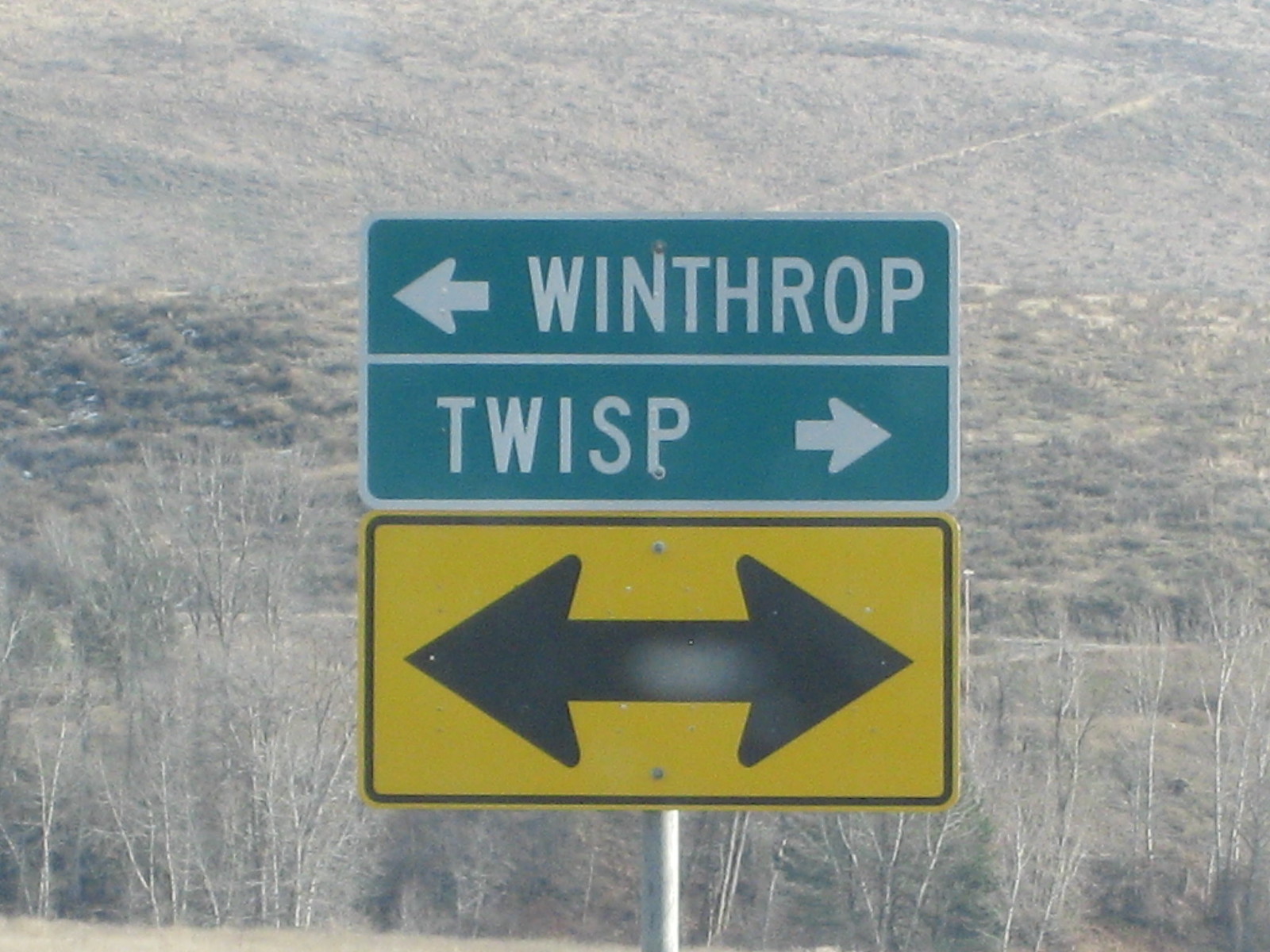The photograph captures a roadside scene featuring two prominent road signs and a dry, barren landscape stretching into a valley. In the foreground, the grass appears very dry and yellowish, with dormant, leafless trees and bushes scattered around. Mounted on a circular metal pole, the two street signs are stacked vertically. The top sign is green with white text, indicating "Winthrop" with an arrow pointing left and "Twisp" with an arrow pointing right. The sign is split in the middle by a white line. Below it is a yellow sign outlined with a black border, displaying black arrows pointing in both directions. In the background, a slight path can be seen winding up a hill towards the upper right, providing depth to the scene.